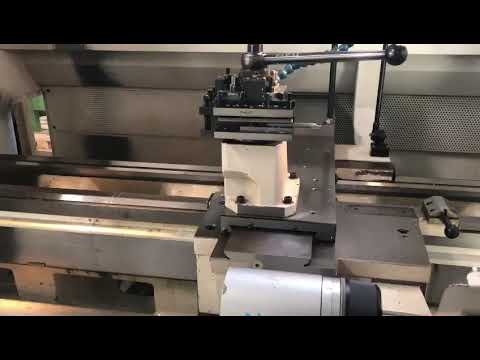The image features an industrial machine centered within a horizontally aligned rectangular frame, bordered by thick black bars at the top and bottom. The machine appears to be a heavy-duty press, evident by its robust construction and multiple metal components. At the top of the machine, a long, horizontal silver bar extends, ending in a black knob, hinting at a mechanism operated by rotating the bar. Below this, the apparatus incorporates several interconnected metal layers, solidified onto a white base with three prominent bolts. This white base sits atop a larger rectangular silver base, suggesting a stable foundation. To the right, another smaller black handle is visible. The machine seems designed for industrial use, likely to press or manipulate materials. Directly behind the machine, a conveyor belt-like strip runs perpendicular to it, enhancing the industrial setting. The black borders at the top and bottom add a defined framing to the image, which solely focuses on the machinery, as no floor, walls, or people are visible.